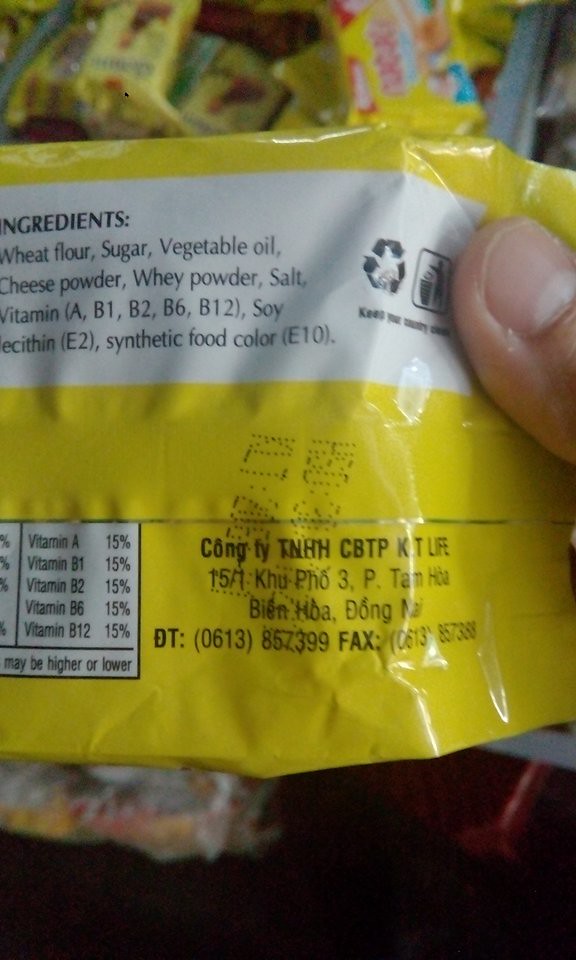In this vertical, dimly-lit photograph, a person is holding a yellow bag of food with their thumb visible on the right side of the image. The bag is displayed from the back, revealing its list of ingredients printed in black lettering against a white background near the top. Ingredients such as wheat flour, sugar, and vegetable oil are legible. Towards the right side of the bag, there's a black recycling icon. Above the yellow bag, other similar bags with blue and red designs are partially visible, adding more colors above the main focus. The area below the yellow bag fades into darkness, obscuring further details. The yellow bag itself is notably wrinkled, and near its bottom, text that seems to include an address is printed in black letters.